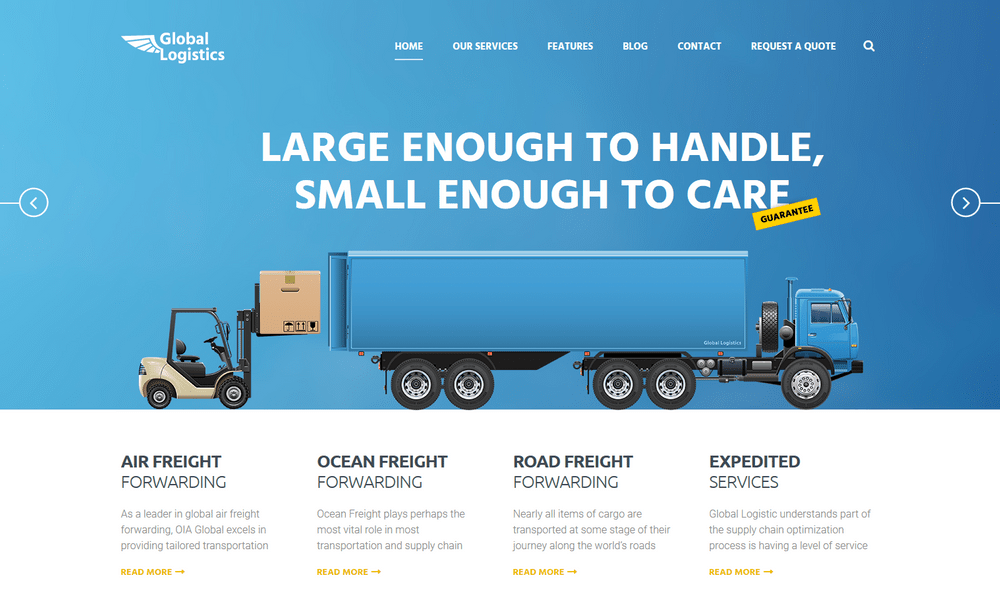The web page from the company Global Logistics prominently features the name "Global Logistics" in white text at the upper left-hand corner, accompanied by their logo—a white, extended wing. The top navigation bar, also in white, includes options for Home, Our Services, Features, Log, Contact, Request a Quote, and a magnifying glass icon for search. Below this, in bold white capital letters, the tagline "LARGE ENOUGH TO HANDLE, SMALL ENOUGH TO CARE" is displayed against a bright blue background. The word "care" is accented with an orange banner containing the word "GUARANTEE" in black text. The central image shows a vibrant blue semi-truck with a mechanical vehicle unloading a large box from its back. The entire image maintains a bright blue backdrop. Beneath this, on a white background, various service categories are listed from left to right: Air Freight Forwarding, Ocean Freight Forwarding, Road Freight Forwarding, and Expedited Services.